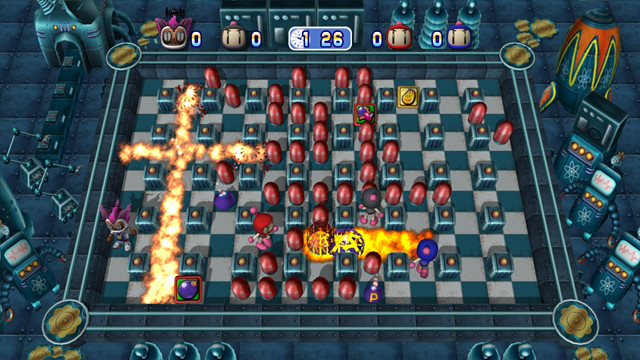This is a detailed screenshot from a classic Bomberman series video game. The scene is viewed from a slightly tilted bird's-eye perspective, showcasing a checkerboard-style game board with alternating white and teal tiles. The board is maze-like, resembling a labyrinth with five rows and eight columns, punctuated by red obstacles blocking various paths. 

At the top of the screen, there are images of four different Bomberman characters with zero scores next to their faces—one character dressed in blue, another in red, the third in black, and the last in pinkish-purple. Centrally positioned above the characters, a clock displays the time "126". 

The game appears chaotic, with yellow and red cross-shaped explosions visible on the board potentially hindering the players' paths. The characters, depicted in a pixelated, cartoonish style, seem to be navigating the maze while avoiding or triggering bombs to outmaneuver each other. Surrounding the game board, robots with lifeline-like displays on their screens add an industrial feel to the game, suggesting a factory setting. The players are probably trying to eliminate each other through strategic bomb placement to emerge victorious in this action-packed, multiplayer game scenario.